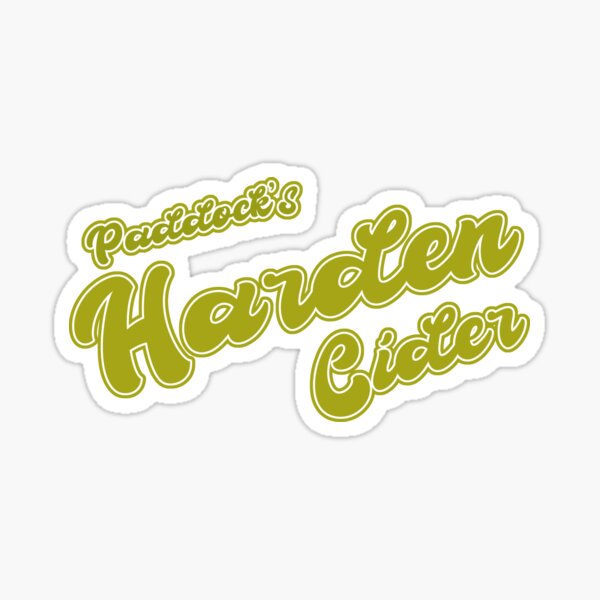The image features a square label for "Paddock's Harder Cider" prominently displayed against a bright white background. The label itself has a greenish lime color with large, fancy cursive letters. "Paddock's" is written at the top, "Harder" is angled across the middle, and "Cider" is at the bottom, with each word on a separate line. The text appears in stylized bubble letters, all connected, and outlined first in white and then in a pale yellow-beige color. The entire label is encompassed by a whimsical cloud-like border, traced in a soft blue that loops around each word, giving the appearance of a continuous flowing design. The label, centered in the image, resembles a meticulously crafted sticker or logo, adding a playful yet elegant touch with its angled and ornate lettering.